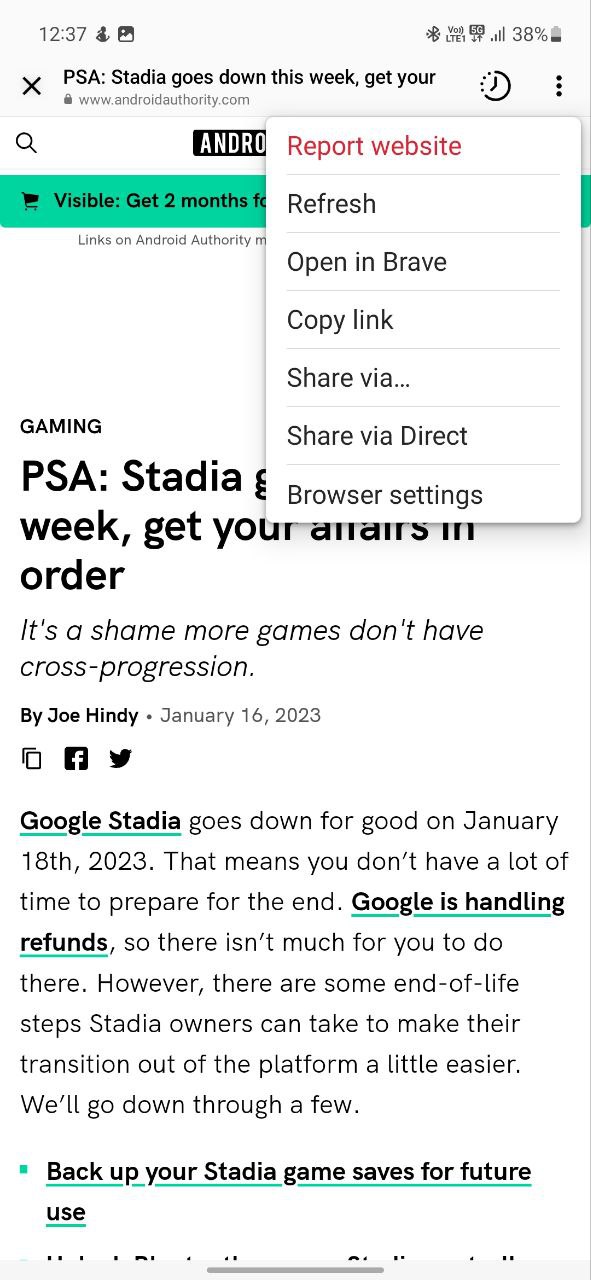**Detailed Caption:**

In this screenshot taken from an article on Android Authority, the device display at the top shows a time of 12:37, a 5G internet connection, and a battery level of 38%. The primary focus of the image is an article headline that reads, "PSA: Stadia goes down this week, get your affairs in order." A notification box partially obscures the content, with options to report the website, refresh, open in Brave, copy the link, and share via various methods. 

Behind this notification box, there is a partially visible advertisement for a mobile service stating, "Visible: Get two months free," although the rest of the text is obscured. The article, authored by Joe Hindi and dated January 16th, 2023, explicitly warns that Google Stadia will be shutting down permanently on January 18th, 2023. This means users have a limited time to prepare for the closure. 

The article mentions that Google will be handling refunds, suggesting that there isn't much for users to do in that regard. However, it does provide steps for Stadia owners to ease their transition from the platform, such as backing up their game saves for future use. Additionally, there are Facebook and Twitter share icons present beneath the introductory content. 

Overall, the image underscores the urgency for Stadia users to take action before the imminent shutdown, while navigating through overlapping notifications and partially occluded text.